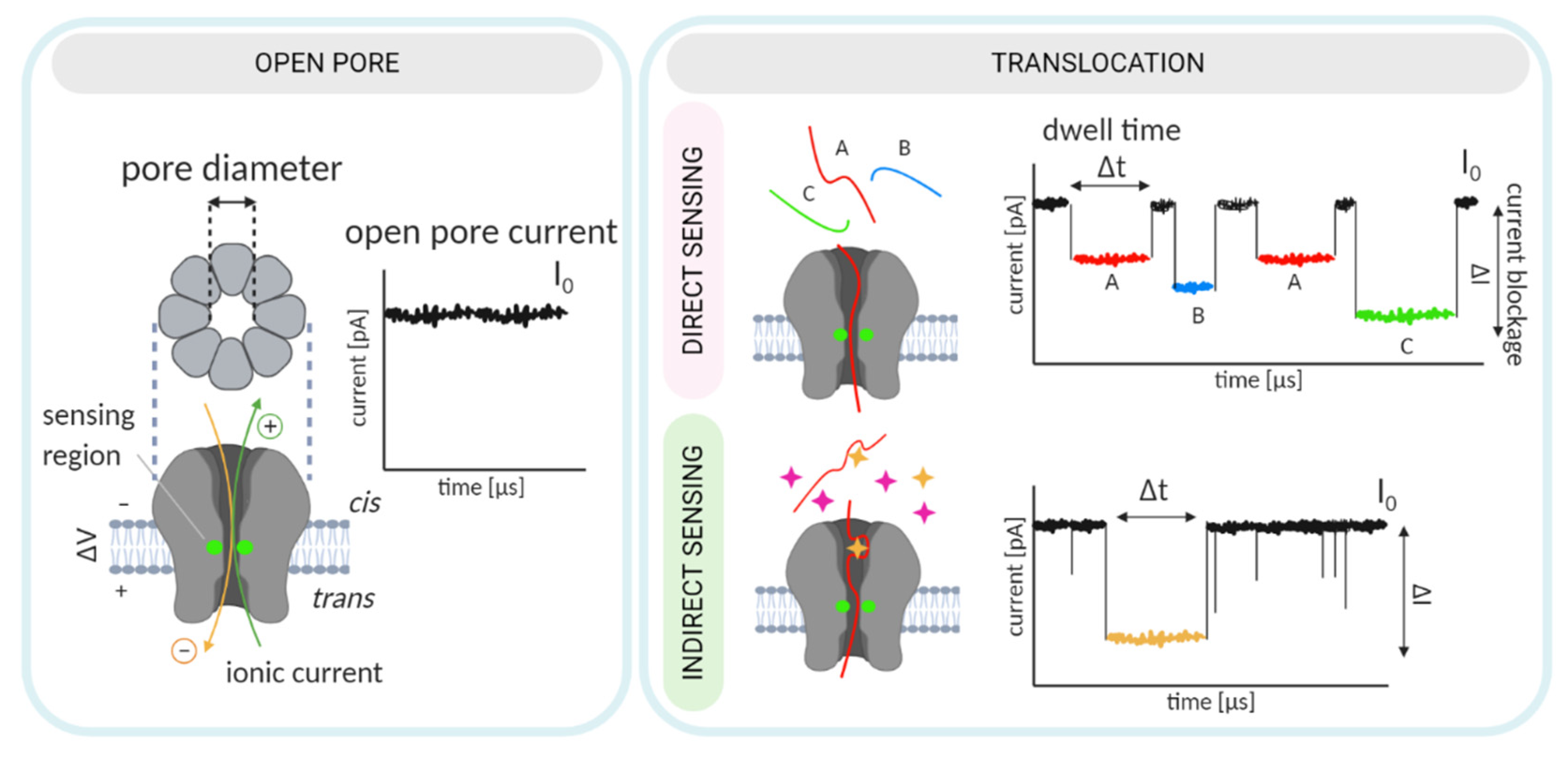The image is a detailed graphical representation of the human nervous system at a microscopic level, showcasing the flow of ionic currents through a transmembrane protein embedded in a phospholipid membrane. The diagram is bordered by a square blue frame, with a wider rectangular blue box on the right labeled "translocation."

In the central portion, various technical terms are highlighted, such as "pore diameter," "sensing region," "ionic current," "open pore current," and "translocation." The illustration features a tooth-like transmembrane protein, indicating a complex interaction across the phospholipid membrane, which consists of hydrophilic heads and hydrophobic tails.

Three different models, labeled A, B, and C, are represented by red, blue, and green lines, respectively. These lines are plotted on graphs to show their relation to "open pore current" and "time," with C depicting the lowest current over the longest time. Other elements in the image include labels like "direct sensing" and "indirect sensing," "dwell time," and "current blockage," all critical to understanding the ionic flow and various sensing mechanisms depicted.

A pink bubble in the illustration highlights "direct sensing," whereas "indirect sensing" is indicated at the bottom. A graph on the left illustrates steady-state current over time, while another graph shows variations with a yellow squiggly line that represents changes over time. The overall image offers a densely packed, multidimensional view of neural current sensing and translocation mechanisms.